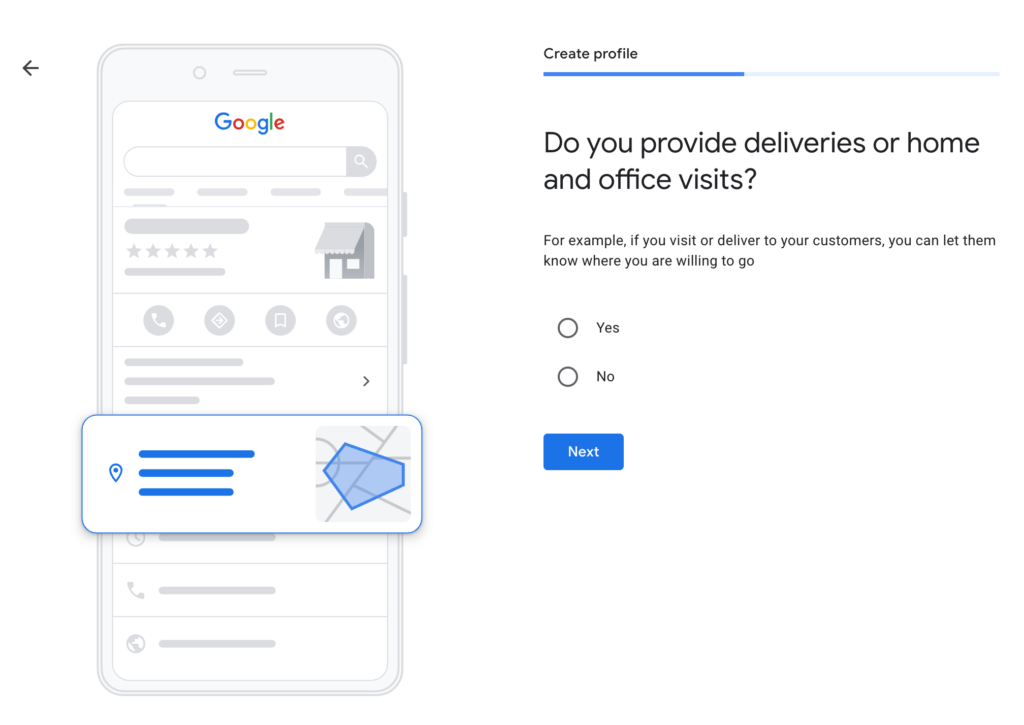The image depicts a detailed view of a cell phone screen against a white background. On the left side of the image, the cell phone screen prominently displays the Google logo at the top, followed by a search bar below it. Centrally positioned on the screen is a pop-up window resembling a map location interface. To the right of this map-like display, there is a crucial Yes or No question: "Do you provide deliveries for home and office visits?" This question is aimed at gathering information regarding the delivery services offered by the user. Beneath the Yes and No options lies a blue "Next" button, which is meant to proceed to the next step. The screen's layout suggests that the user is in the process of setting up a Google profile, specifically relating to delivery services, as Google seeks to confirm whether the user offers deliveries for home and office visits. All text on the screen is black, standing out clearly against the white background.